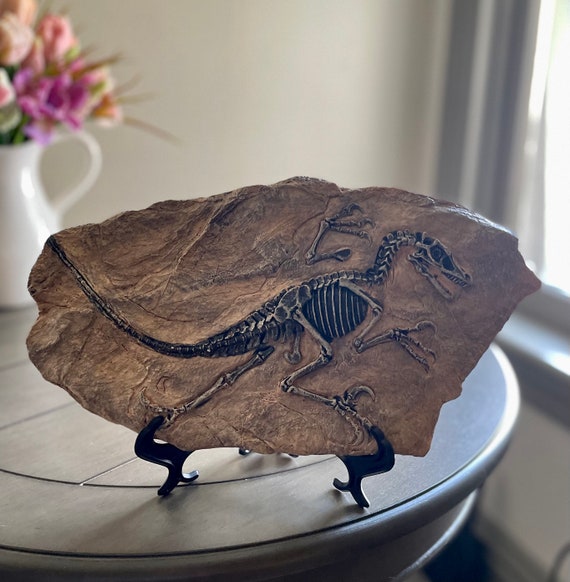The photo features a detailed fossil of a small dinosaur, possibly a velociraptor, encased in a light brown rock. The fossil appears stylized, depicting the dinosaur in mid-run with its sharp claws prominent. This intriguing piece is carefully propped up on wooden legs and placed on a circular end table, suggesting it could be from a museum or a private collection. In the background, a beige wall and a window allowing sunlight to stream in can be seen, enhancing the ambient setting of what appears to be a living room. Complementing the scene is a pitcher with vibrant pink flowers located in the upper left corner, adding a touch of color and warmth to the space.